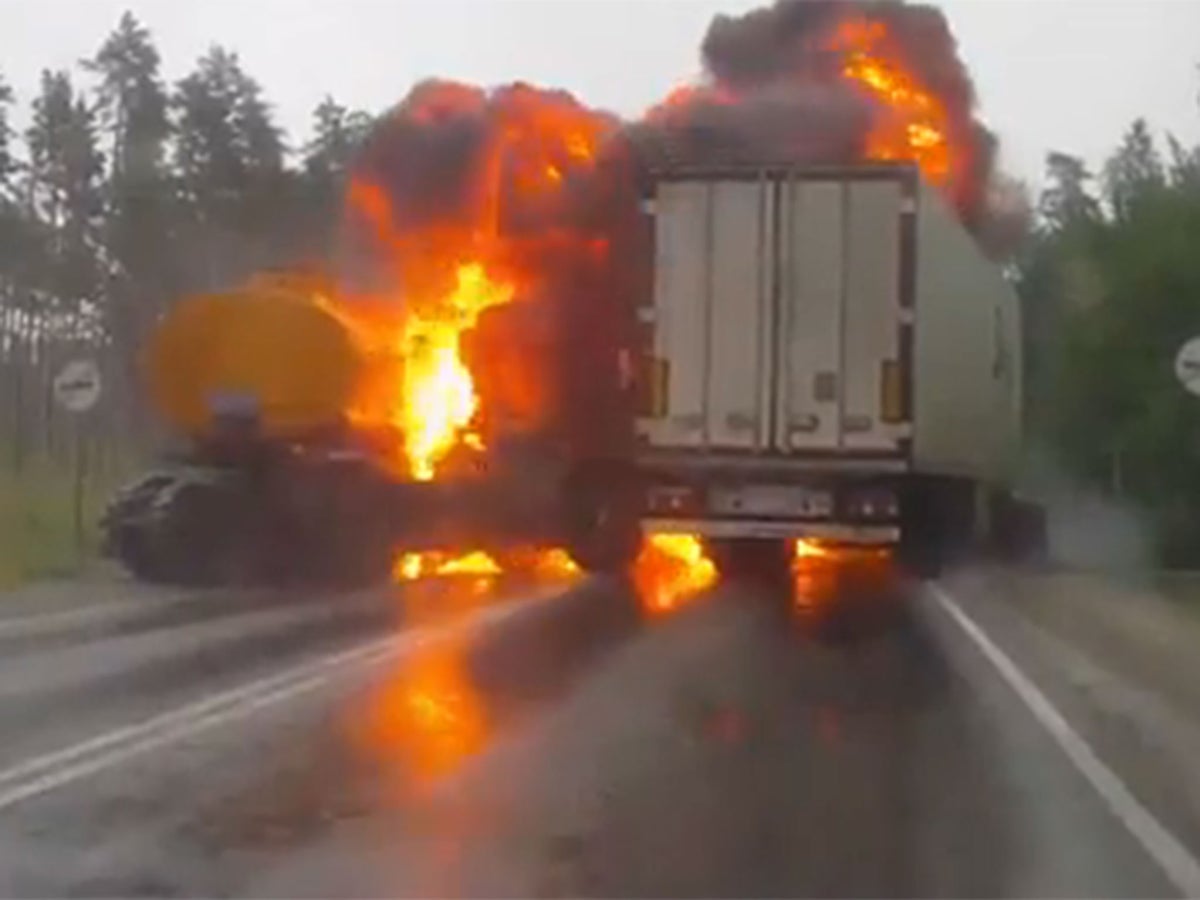A dramatic scene unfolds in this image, capturing the aftermath of a severe collision. At the very bottom, the gray asphalt road is visible, marked by a white line on the right delineating the edge of the lane, and two solid white lines in the center that divide the lanes. Dominating the foreground is the back end of a white 18-wheeler truck, which appears to be involved in the incident.

To the left of the truck, intense orange flames and thick, billowing black smoke indicate a significant explosion, likely resulting from the crash. The blurry silhouette of another black vehicle is partially visible in the left lane, adding to the chaotic scene. 

Surrounding the road are green trees, their foliage untouched by the destruction below. Above, the sky is a light gray, offering a stark contrast to the drama happening on the ground. The image captures a moment of high tension and danger, framed by the serene natural landscape.